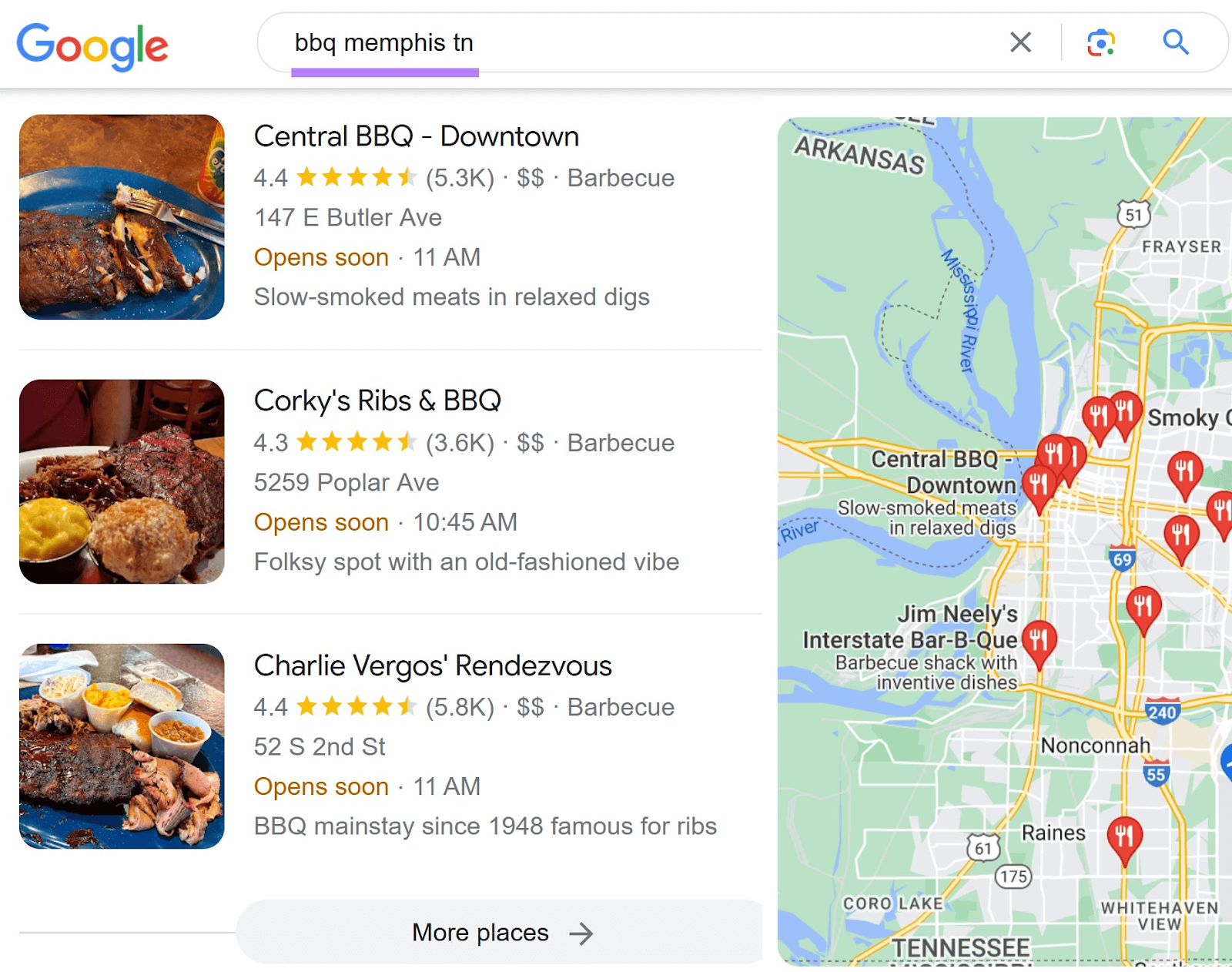The image displays a Google search results page dedicated to "BBQ Memphis Tennessee." In the upper left corner, the iconic Google logo is prominently featured, followed by a search bar containing the keyword query. The left section of the page showcases detailed search results for various BBQ spots in Memphis.

The first listing features a close-up image of succulent ribs on a blue plate, representative of **Central BBQ Downtown**. This entry boasts a 4.4-star rating, notes that it will open soon at 11 a.m., and highlights its offerings of slow-smoked meats in a relaxed atmosphere. The address is also provided.

Immediately below, a second search result highlights **Corky's Ribs and BBQ**, adorned with a picture of ribs alongside various other menu items. This establishment holds a 4.3-star rating and is noted to open soon at 10:45 a.m. It is characterized by its folksy ambiance and old-fashioned vibe.

The third entry showcases **Charlie Virgo's Rendezvous**, also paired with an image of ribs and assorted food on a blue plate. It shares a 4.4-star rating, indicates an opening time of 11 a.m., and acknowledges its historic status in the BBQ scene since 1948, famed particularly for its ribs.

Below these entries is a "More places" button, prompting further exploration of dining options.

Occupying the right side of the page is a detailed map populated with approximately a dozen red pins, each marked with a fork and knife icon to signify restaurant locations. Prominent spots like **Central BBQ Downtown** and **Jim Neely's Interstate BBQ** are among those highlighted on the map.